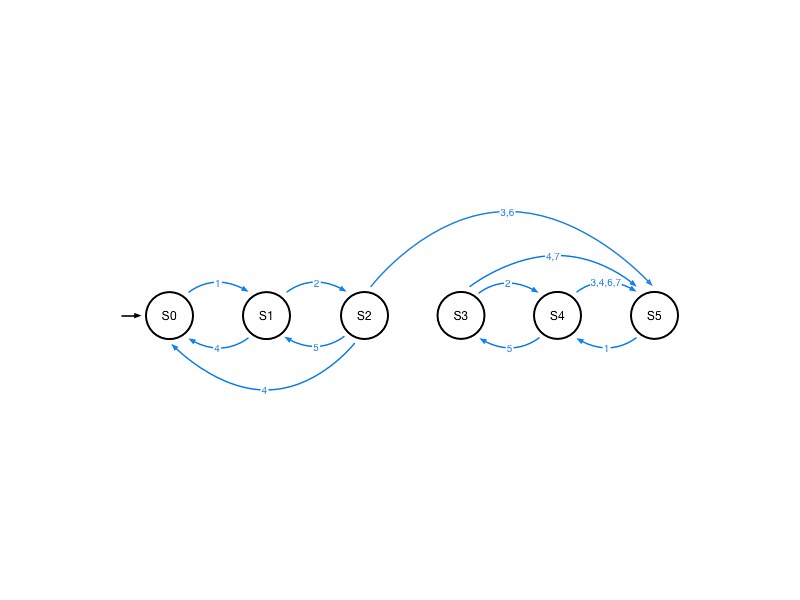This detailed diagram illustrates a series of interconnected steps and states labeled with "S" followed by various numbers, and directional arrows indicating the flow between these states.

1. **Starting Point (S-0)**: On the left-hand side, a black arrow points right to a black circle labeled "S-0".
2. **Transition from S-0 to S-1**: A blue arrow labeled "1" points from "S-0" to another black circle labeled "S-1".
3. **Transition from S-1 to S-2**: From "S-1", a blue arrow numbered "2" guides to a third black circle marked "S-2".
4. **Transition from S-2 to S-5**: A blue arrow labeled "3.6" extends from "S-2" to a circle designated as "S-5".
5. **Transition from S-5 to S-4**: "S-5" has an arrow marked "1" leading to a circle labeled "S-4".
6. **Transition from S-4 to S-3**: "S-4" features an arrow with a "5" pointing to a circle labeled "S-3".
7. **Loop Between S-3 and S-4**: From "S-3", a blue arrow marked "2" returns to "S-4".
8. **Complex Loop involving S-4 and S-5**: "S-4" shows several arrows labeled "3", "4", "6", and "7" pointing back to "S-5".
9. **Additional Arrows from S-2**: "S-2" has another arrow marked "4" leading back to "S-0", and another arrow labeled "5" directing to "S-1".
10. **Arrow from S-1 to S-0**: Finally, "S-1" has an arrow labeled "4" that circles back to "S-0".

The diagram comprehensively maps out a network of pathways between these states, labeled with arrows and numbers that likely represent steps or transitions in a process.